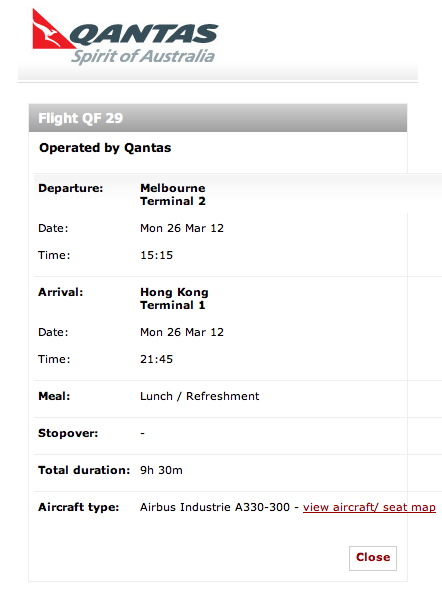The image is a screenshot of a section of a web page, featuring travel details for a flight operated by Qantas, Spirit of Australia. The web page has a clean layout with a white background and black text for readability. 

In the upper left corner, the Qantas logo is prominently displayed. The logo consists of a red right-angled triangle containing an outline of a hopping kangaroo in white, symbolizing the airline's Australian heritage. Adjacent to the logo, the name "Qantas Spirit of Australia" is clearly visible, further emphasizing brand identity.

Below the logo, a grey bar contains the flight number, "Flight 29." 

The main body of the page provides details about the flight in a structured format:

- **Operated by:** Qantas
- **Departure:**
  - **Location:** Melbourne
  - **Terminal:** 2
  - **Date:** Monday, 26th March 2012
  - **Time:** 15:15

- **Arrival:**
  - **Location:** Hong Kong
  - **Terminal:** 1
  - **Date:** Monday, 26th March 2012
  - **Time:** 21:45

- **Meal:** Lunch and Refreshment